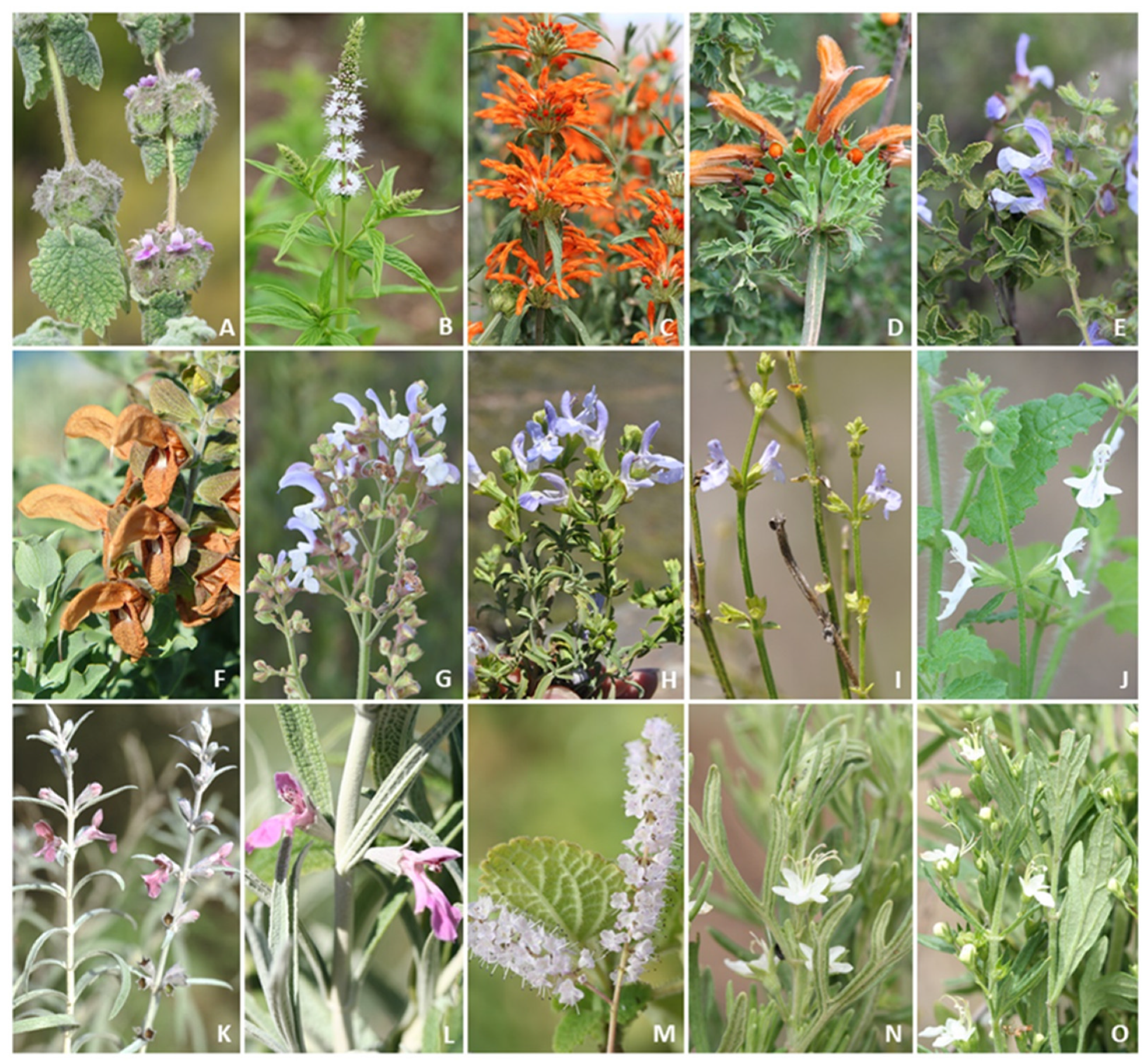The image displays a grid of 15 photographs of various wildflowers, labeled from A to O, positioned within a 3x5 layout. Each label is situated at the bottom right corner of each picture. The photos feature close-up shots of diverse flowering plants, showcasing species that likely thrive in natural, wild environments rather than cultivated gardens. The colors of the flowers vary widely, including bright oranges, pinks, purples, and whites, with green stems and leaves in the background. For example, picture A has a pink flowering plant, while B and J feature white flowers; C and D show orange blooms. E presents a purple flower, and H through I and part of M to O include shades of lavender and white. The greenery is common across all photos, with some plants, like those in images J and O, displaying white buds that are on the verge of blooming. This assortment of flora, perhaps sourced from a hiking trail or documented for a plant identification guidebook, captures the variety and beauty of wildflower species in their natural habitats.